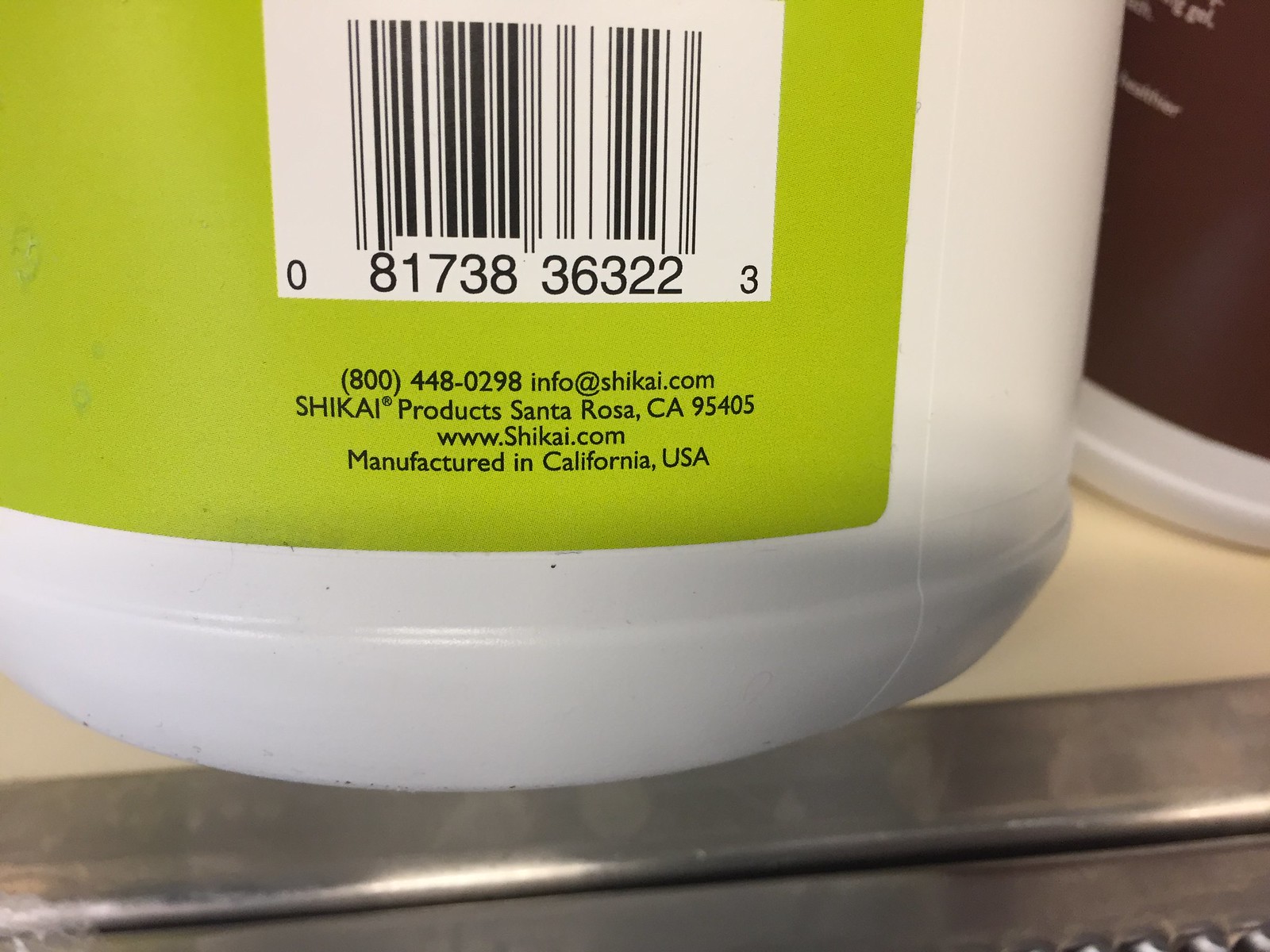The image depicts the back of a white container with a lime-colored background. The container features a label that provides various pieces of information. It includes a phone number and the email address info@shikhae.com. The label identifies the brand as Shikhae Products, located in Santa Rosa, California, complete with a zip code. The website for Shikhae Products is also listed, and the label states that the product is manufactured in California, USA.

The container appears to hold a liquid, although it could be the bottle itself giving this impression. The label also includes a barcode. Additionally, there is a reflective silver section in the image, which might be a conveyor belt, suggesting the scene could take place in a store, particularly at the checkout area. Next to the featured container, there is a brown container, implying the presence of shelving and reinforcing the notion that the setting is a retail store environment.